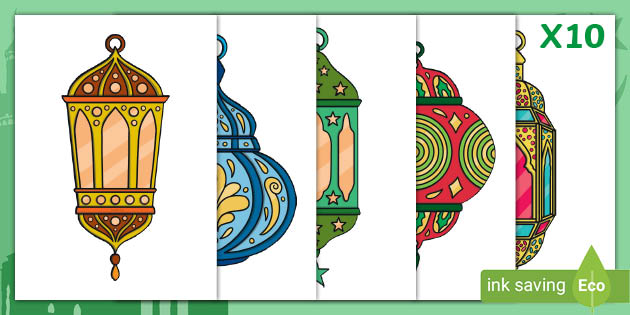The image displays a series of staggered and overlapping colorful cartoon depictions of lanterns or wall sconces, each designed with a Middle Eastern stained-glass style theme. The leftmost lantern is shown in full, featuring a decorative hanging hook, a triangular top section divided into three parts, and a rectangular body adorned with small beads and glass panels. The subsequent lanterns are partially covered by the ones to their left. The second lantern, visible around halfway, depicts a more bulbous shape in dark blue, light blue, and yellow tones. The third lantern showcases various shades of green, while the fourth combines red, green, and yellow hues with star-like beads. The final lantern is broad in the mid-section and ornate, featuring pink, yellow, and blue colors. The entire design is framed with a green border. In the top corner, the text "X10" is displayed, and in the bottom corner, a green box labeled "ink saving" with a green leaf icon stating "eco" emphasizes the environmentally friendly nature of the depicted items, suggesting it might be an advertisement for a printer.